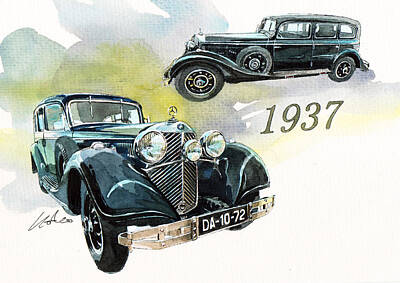The image is a watercolor painting with a beige background adorned with random pastel splashes of green, blue, and purple. It showcases two antique Mercedes Benz cars, primarily depicted in blacks and subtle greys. The top car is viewed from the side, while the bottom car, in the lower left, is presented from a front-angle perspective, slightly off to the side. Both cars feature distinct characteristics including three round headlights, running boards, spare tires, and large headlights. One notable detail is the black license plate that reads DA-10-72, prominently displayed on the front bumper of the larger car. The year '1937' is written in black in the middle of the image, hinting at the cars' era. Additionally, there is an artist's signature on the left side below the depiction of the cars, indicating the creator of this greeting card-like, nostalgic illustration.